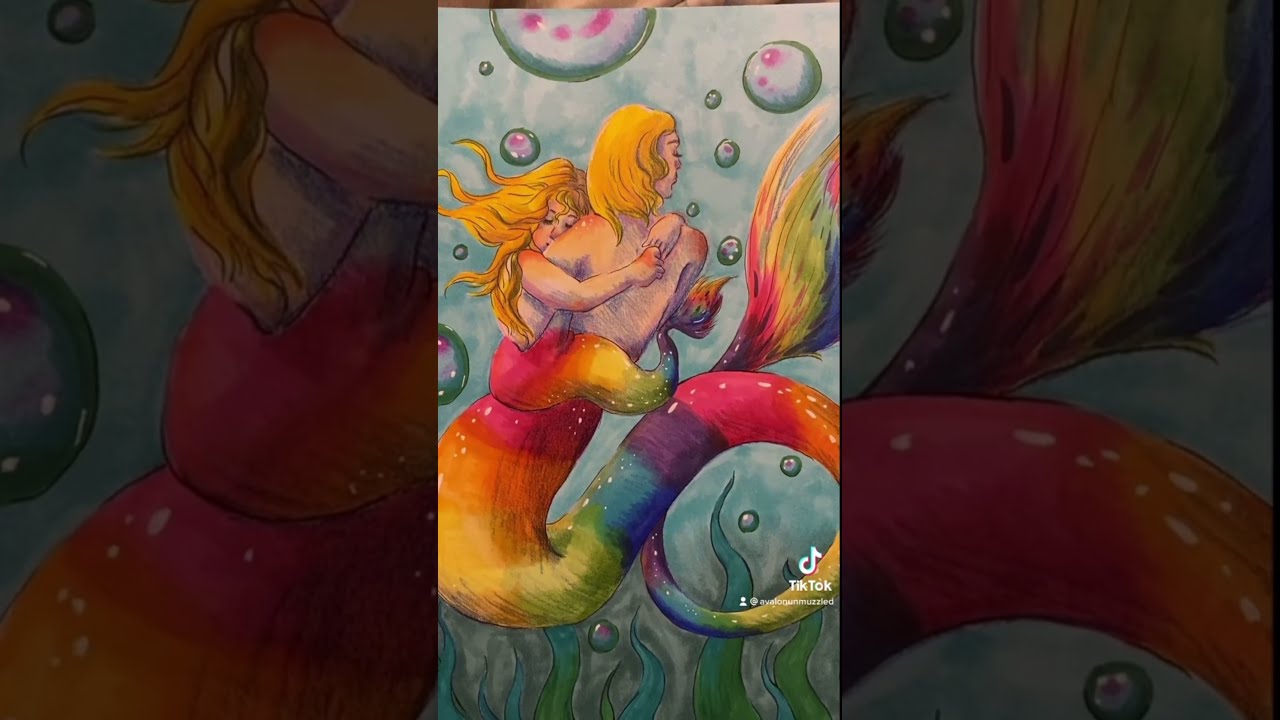The image is a vibrant and whimsical drawing divided into three vertical sections. The central section showcases a captivating underwater scene with two mermaids, a smaller one appearing to be asleep in the embrace of an adult mermaid. Both mermaids have cream-colored skin and flowing yellow hair, while their tails gleam with the full spectrum of rainbow colors—red, orange, yellow, green, blue, and purple. Surrounding them are numerous bubbles, indicative of their oceanic habitat, which is bathed in shades of blue. At the bottom of this aquatic world, green seaweed sways gently. The first and third sections of the image consist of darkened close-ups of the main scene. In the bottom right corner, the image bears a TikTok logo with the handle "@AvaloGunMuzzled" written below. The overall style of the image is distinctly cartoonish and artistic, suggesting it is a screenshot taken from a TikTok video.